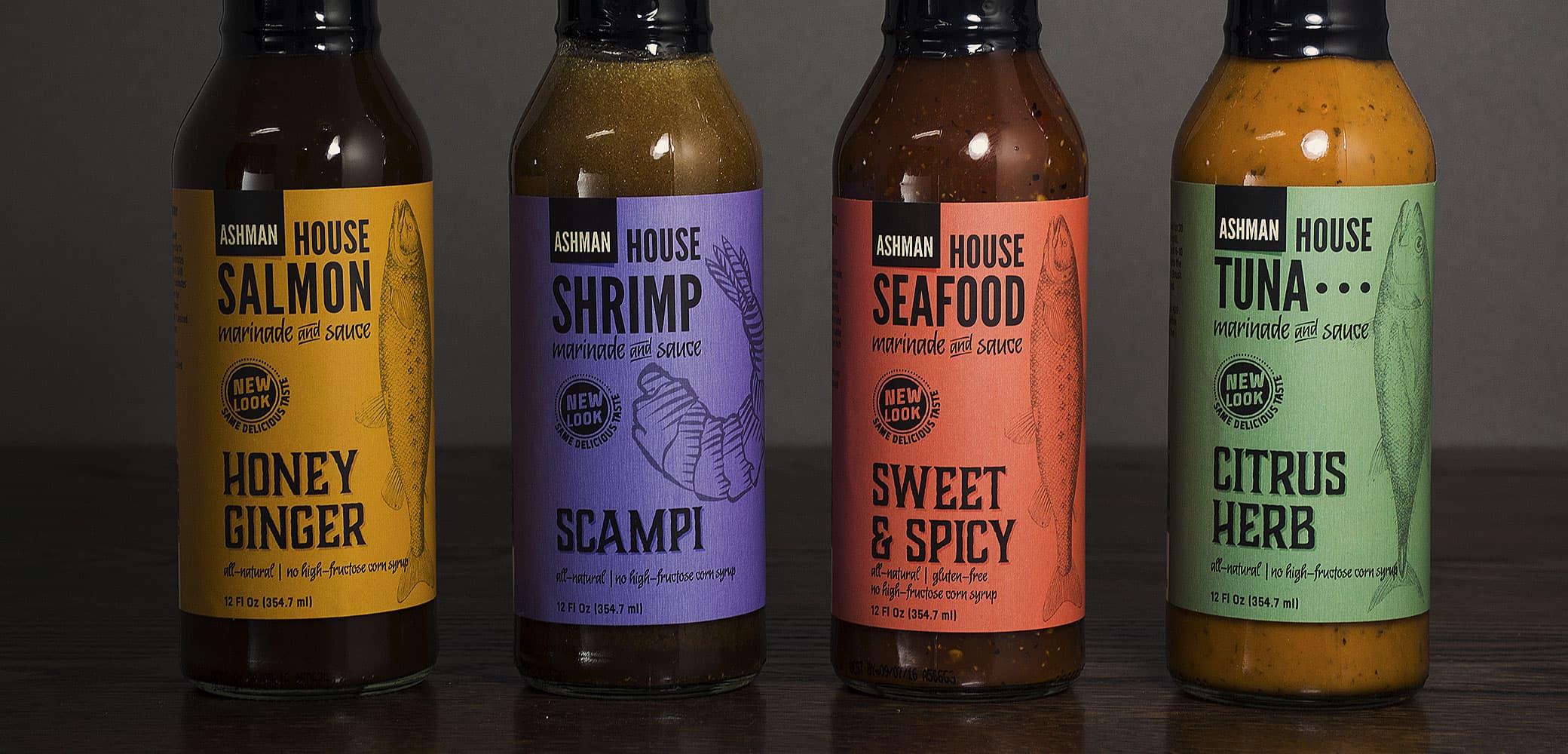This photograph features a close-up of four glass bottles filled with various sauces, neatly lined up side by side on a dark wooden table with a reflective surface. The background is a gray wall, providing a neutral backdrop for the vibrant labels on the bottles.

From left to right:

1. The first bottle has a yellow label that reads "Ashman House Salmon Marinade and Sauce. New Look, Honey Ginger, 12 fluid ounces." It includes an image of a salmon.
2. The second bottle features a bluish-purple label that states "Ashman House Shrimp Marinade and Sauce. New Look, Scampi, 12 fluid ounces," accompanied by an image of a shrimp.
3. The third bottle boasts a pinkish-red label with the text "Ashman House Seafood Marinade and Sauce. New Look, Sweet and Spicy, Gluten-Free, 12 fluid ounces," displaying an image of a fish.
4. The fourth bottle is adorned with a green label that says "Ashman House Tuna Marinade and Sauce. New Look, Citrus Herb, No High Fructose Corn Syrup, 12 fluid ounces," featuring an image of a tuna fish.

Each bottle is transparent, allowing the sauces inside to be visible, and they are topped with black caps.